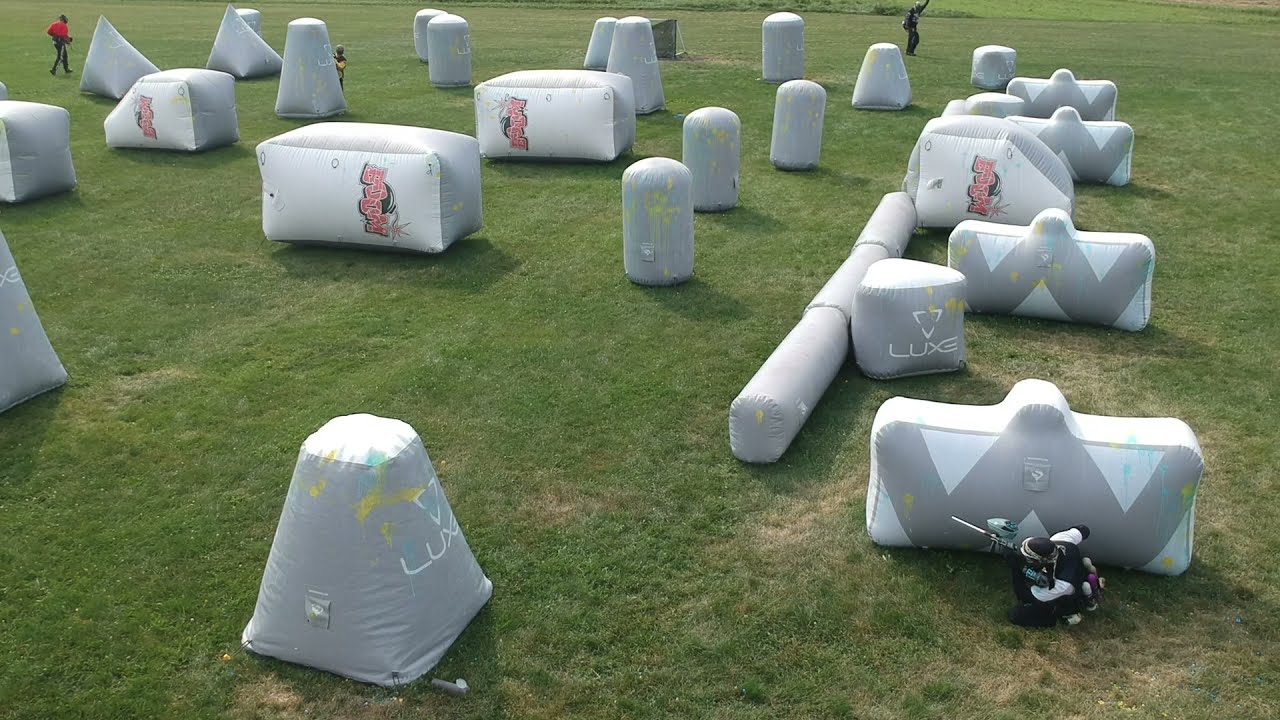This is a dynamic photograph taken outdoors during the daytime, capturing an intense game of laser tag with paintball elements. The game is set on an expansive, well-trimmed grass field, possibly AstroTurf, which provides a vibrant green backdrop. The field is cluttered with a variety of inflatable obstacles of different shapes and sizes, reminiscent of tackle dummies at NFL training camps, and including a mix of pyramidal and rectangular structures covered in paint splatters.

In the lower right-hand corner, a player is seen crouched behind a W-shaped inflatable obstacle. This individual is equipped with a black paintball helmet, a black vest over a white long-sleeve shirt, and a paintball gun with a blue canister. Additional canisters in white and purple are strapped to his back, indicating he's well-prepared for the match. Across the field, three more players are positioned: two in the upper left-hand corner and one in the upper right-hand corner, the latter of whom appears to be walking away, possibly indicating he has been tagged out. The overall scene exudes a high-energy, tactical atmosphere as players utilize the geometric inflatables for cover amidst the flat, green playing field.